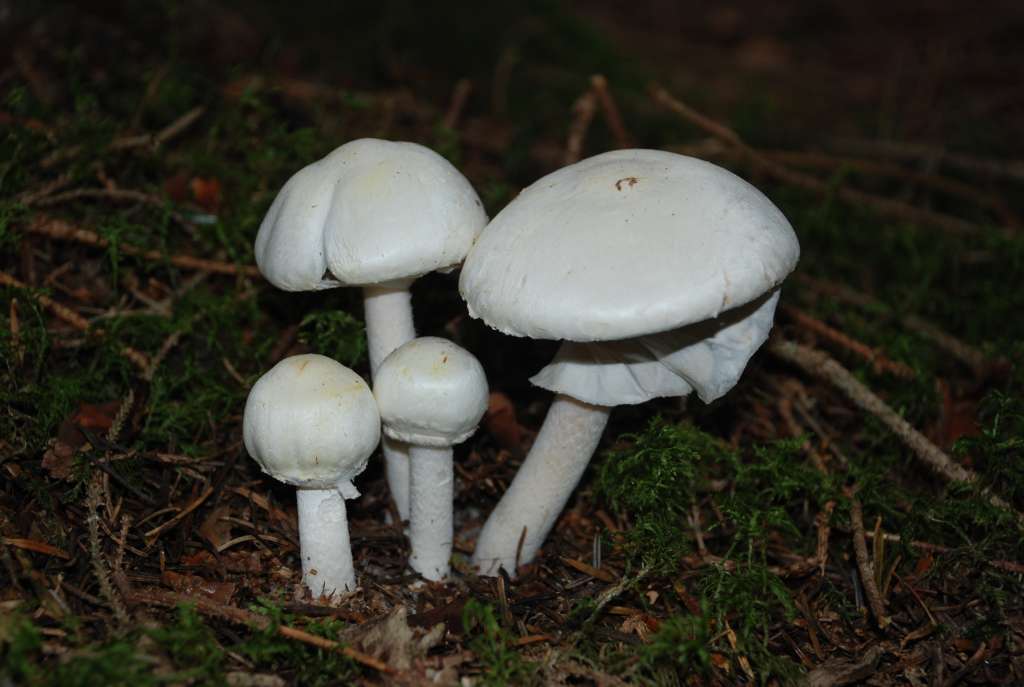In the center of this nighttime photo, four white Agaricus abruptibulbis mushrooms, also known as bulbous flat bulb mushrooms, emerge from the forest floor. The image, illuminated by a flash, captures the dark, out-of-focus background interspersed with patches of green grass, dirt, tiny sticks, and fallen leaves. 

On the left, two smaller mushrooms with short white stems and round caps display subtle brown smudges on their tops. Behind them, a medium-sized mushroom stands taller, its cap noticeably larger. To the right, a large mushroom, equal in height to the medium one but with a cap twice the diameter, features a distinctive brown spot shaped like an 'N' and slight greenish-yellow smudges. The largest mushroom also exhibits a skirt-like tissue under its cap, resembling delicate tissue paper. 

This dark, detailed composition highlights the intricate textures and subtle nuances of these fascinating nighttime fungi.